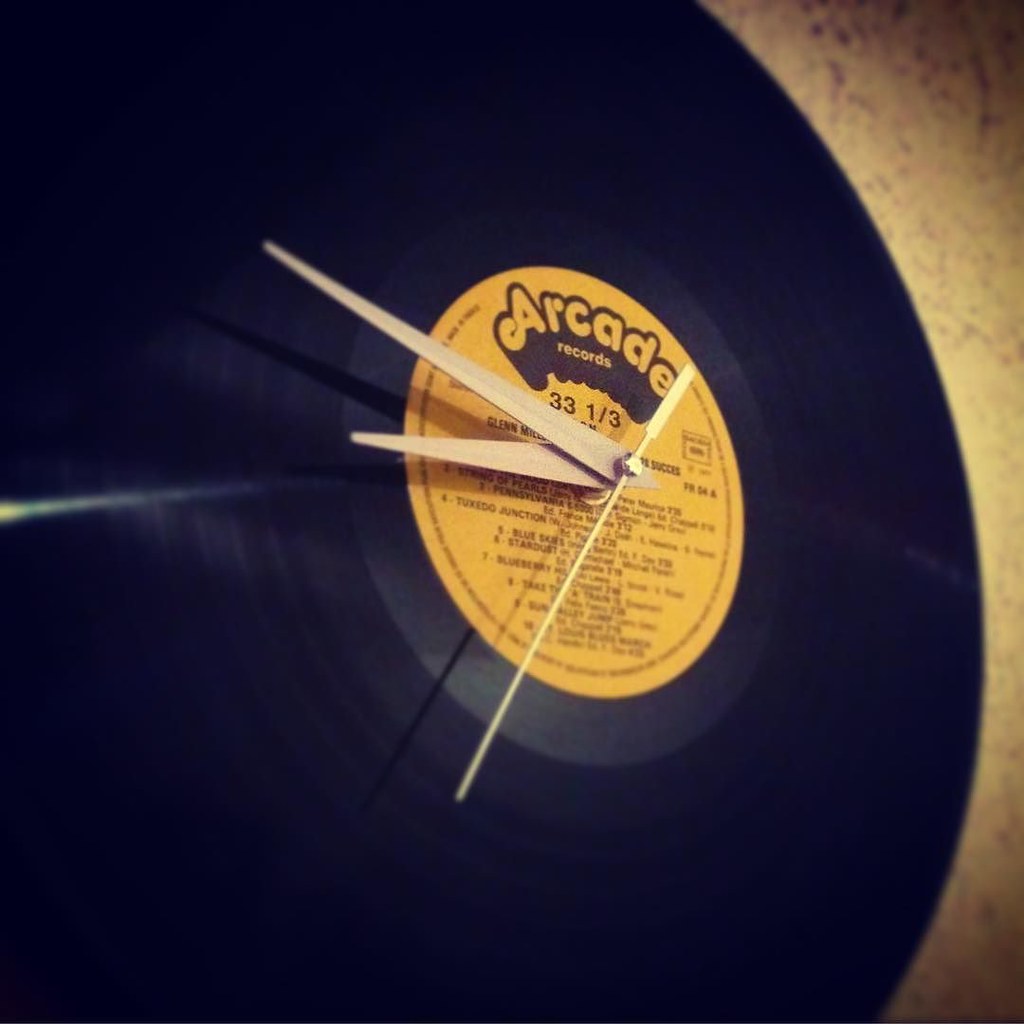In this photograph, we see a unique clock made from a vintage black record, prominently displayed on a wall. The record, crafted by Arcade Records, features the Glenn Miller Band and includes the tracks "Tuxedo Junction" and "Stardust," though the other song titles are not fully legible. The record-turned-clock is designed with two hour and minute hands, as well as a second hand, showing the time to be approximately 9:50. The clock appears to be a 33 1/3 RPM record, transformed into a timeless wall piece. The photograph is taken from a side angle, giving a partial view of the wallpaper behind it, which remains largely indistinct. This charming and nostalgic artifact serves both as a functional timepiece and a tribute to classic music, making it a perfect addition to any wall.